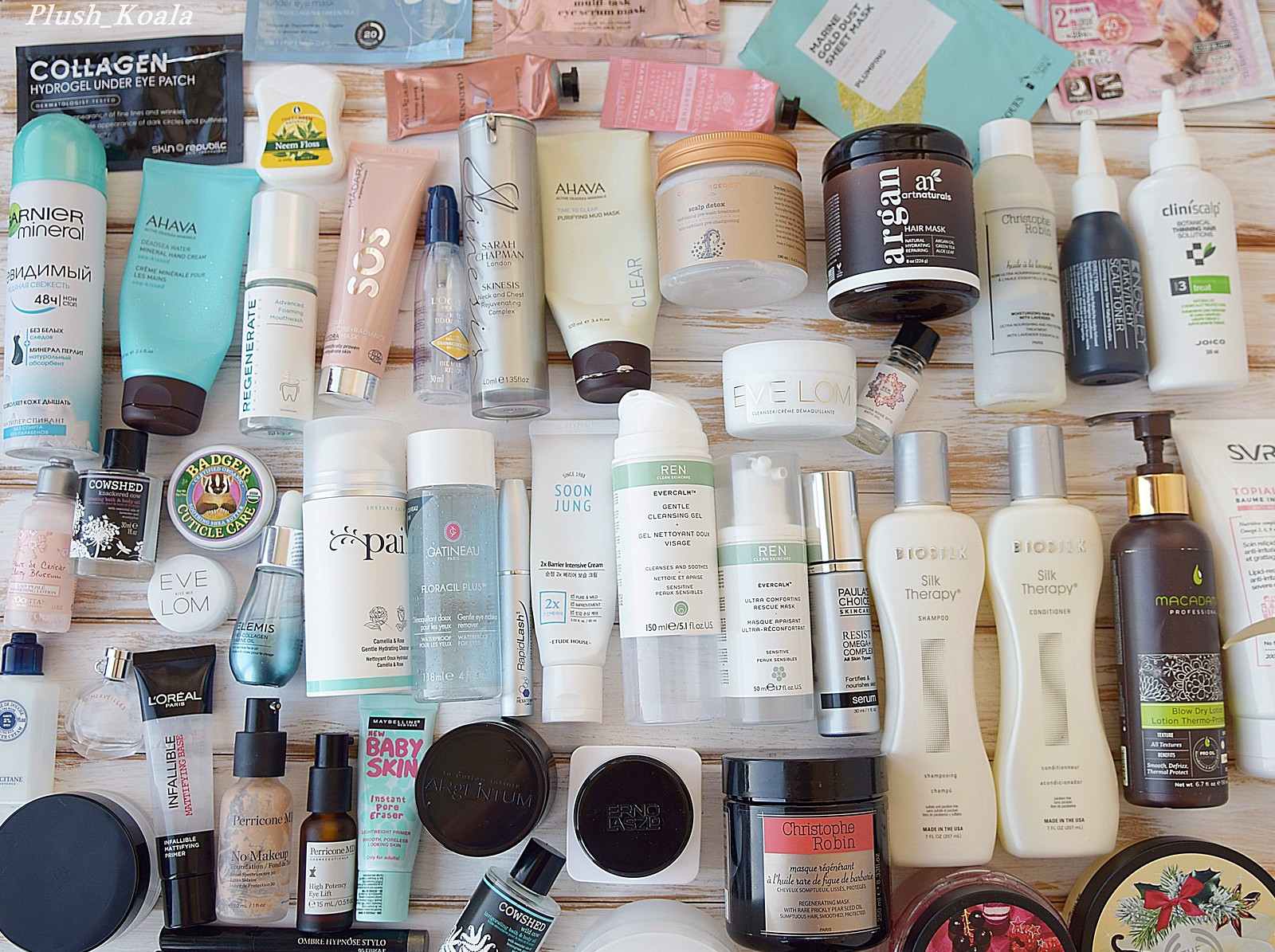The photograph showcases an array of approximately 50 different lotion bottles, meticulously arranged side by side on a wooden table. Each bottle stands independently, ensuring a spacious layout that avoids any overlap or cramping. The bottles exhibit a predominant color palette of white, interspersed with select blue, pink, and black variants, adding a subtle vibrancy to the overall composition. The table itself, painted white, reveals hints of its wooden texture through small, brown carve marks that lend a rustic charm to the scene. In the top left corner of the image, the text "plush_koala" is displayed in a crisp white font, adding an element of branding to the photograph.